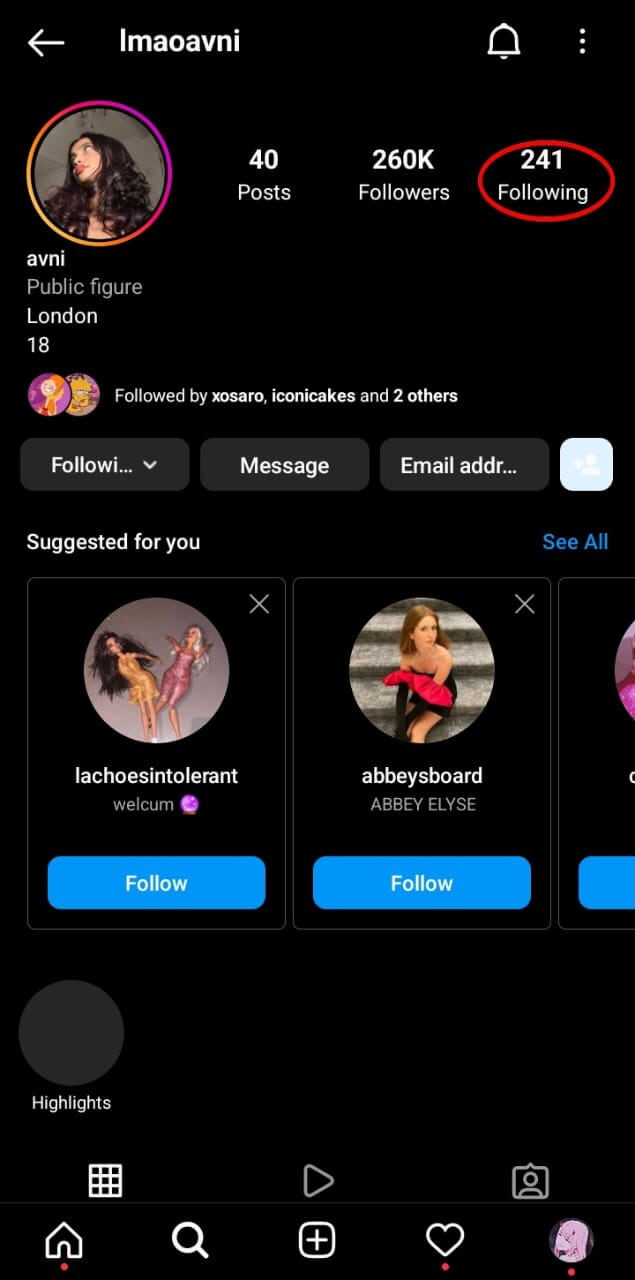This detailed caption accurately describes the elements present in the Instagram screenshot:

---

A detailed screenshot of an Instagram profile is depicted. The background is pitch black with a view of the top-left corner. A white arrow pointing left is visible, accompanied by the text "I M A O A V N I" in bold, black capital letters. To the right, a gray-bordered, black interior bell notification icon is present, followed by three vertically-aligned gray dots.

On the left side of the screen, there's a circular image that transitions from violet at the top, to red in the middle, and orange at the bottom, blending slightly with red. The picture within the circle features a girl with long black hair draped past her shoulders, looking up and to the left. Behind her, the ceiling appears white.

To the right of her image, in large bold white text, the number 40 is displayed, indicating the number of posts. Adjacent to this, "260K" denotes the number of followers, while "241" indicates the following count, all encircled by a red outline.

Below the main profile picture, the text "A V N I" is displayed in white, followed by "Public Figure" and "London 18". There are two small profile pictures next to it, one unidentifiable cartoon character and another belonging to someone named Lisa. The text "Followed by [name] and [another name] and 2 others" appears below these images.

Three gray tabs with white lettering are showcased below: "Following," "Message," and "Email." Further down, the section "Suggested for you" is in white, with a blue "See All" to the right. Two profile suggestions follow, each with a picture, name, and a blue "Follow" button; the edge of a third suggestion is partially visible.

A gray circle labeled "Highlights" is positioned below, adjacent to icons including a calendar, a triangle pointing right, and a profile icon within a square. At the bottom of the screen, the traditional navigation bar features a home icon with a red dot, a search icon, a square with a plus sign, a heart icon with a red dot, and a profile picture of a pink animal cartoon, also marked with a red dot.

---